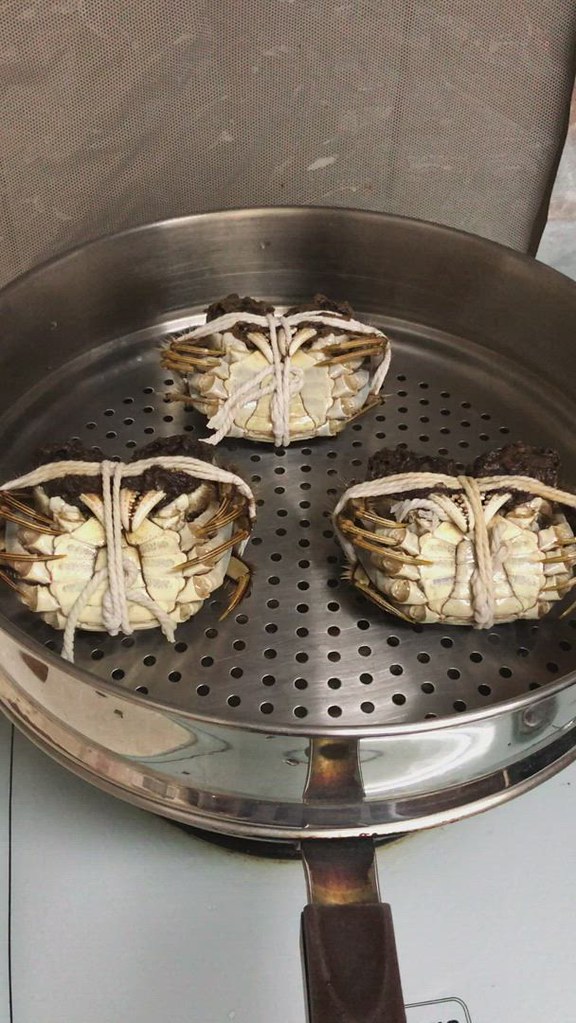In this detailed color photograph captured in portrait mode, we see a close-up of three blue crabs positioned upside down in a round metal steamer pan with deep sides and a perforated bottom, suggestive of ongoing cooking. The pan rests on a white stovetop with parts of the countertop, possibly marble, visible in the frame. The crabs, arranged in a triangular shape and not touching each other, are bound securely with light brown or white twine around their middle. Their claws are folded over their undersides, and the stuffing inside them appears dark brown in color. The pan also features a handle with a black plastic grip, extending towards the bottom of the image.